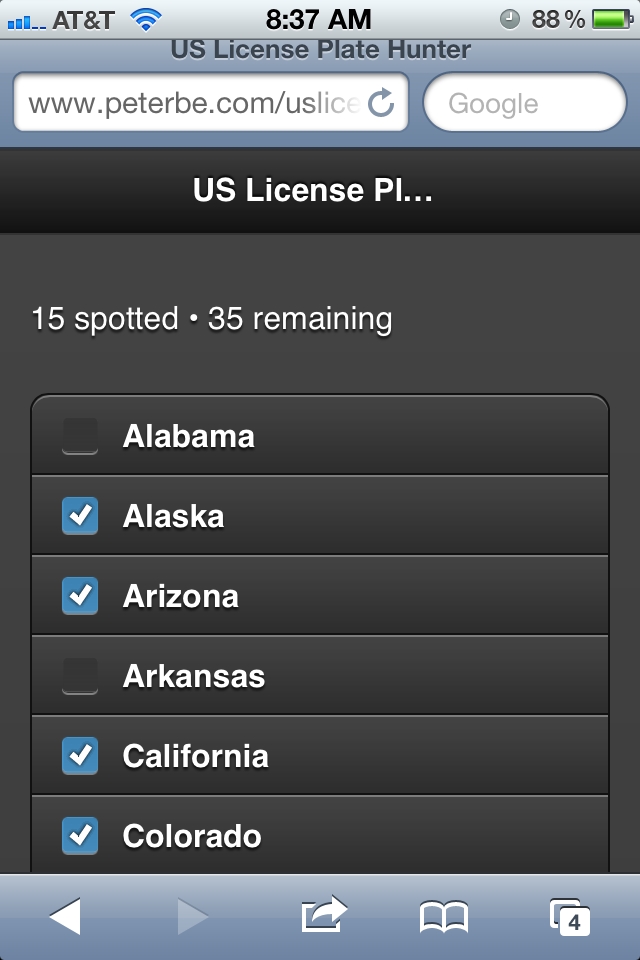The image shows a smartphone screen with the current time displayed as 8:37 AM and the battery level at 88%, serviced by AT&T. The top left corner exhibits signal strength bars for both cellular and Wi-Fi connections. 

The main content of the screen is dedicated to an application or webpage titled "US License Plate Hunter" with the URL partially visible as "peterbe.com/uslicense," which is cut off after "e." The page has a Google search bar at the top, followed by a black navigation bar displaying the truncated title "US License PL..."

Below this bar, there's a tracker indicating "15 spotted, 35 remain," suggesting the user is on a quest to spot license plates from all US states. The states are listed sequentially on gray-colored bands. States such as Alabama, Alaska, Arizona, Arkansas, California, and Colorado have blue squares with white check marks next to them, indicating they have been spotted.

At the bottom of the screen, a blue navigation bar features back and forward arrows, as well as icons possibly representing share, bookmarks, and the number "4," which may indicate that there are four active tabs or windows open, and this is one of them.

The interface appears designed for users to mark off license plates as they encounter them, making it an ideal companion for road trips or license plate hunting enthusiasts.